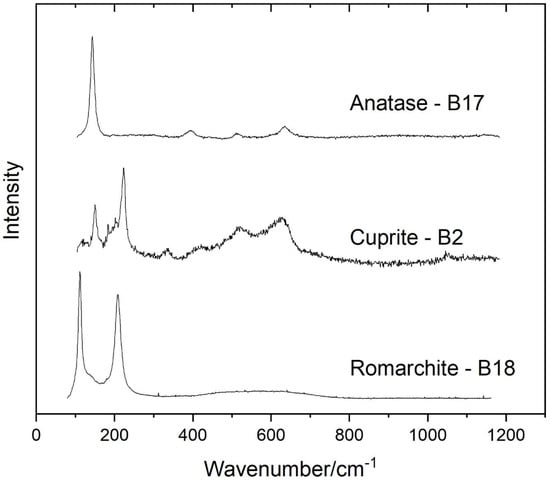The image displays a detailed black and white graph, consisting of three line graphs against a rectangular grid. On the left-hand side, the y-axis is labeled "Intensity," while the x-axis at the bottom is marked with "Wave Number / cm⁻¹." The x-axis runs from 0 to 1,200 in increments, indicated by ruler-like black dashes. 

Each line graph represents different samples. The first line, labeled "Anatase-B17," the second "Cuprite-B2," and the third "Rhomarchite-B18," all feature squiggly lines akin to EKG readouts. Despite variations, all three lines commence with high intensity that decreases and steadies towards the end. The highest peaks nearly reach the 1,200 mark on the x-axis.